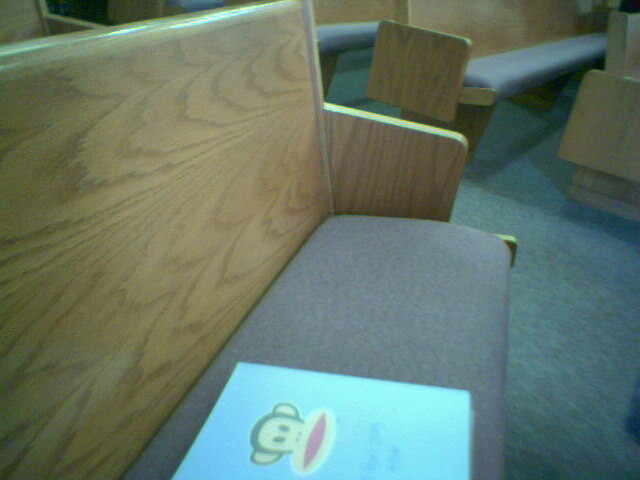This image captures a room filled with pew-like benches, often associated with churches or courtrooms but potentially a meeting or lecture space due to the seating arrangement. The floor is covered in a dusty blue-gray, indoor-outdoor carpet. The benches have sturdy wooden backs and small wooden armrests at the ends, with each seat upholstered in a light slate gray fabric. The photograph is taken from a pew facing left towards an aisle, with additional rows of similar pews visible across the aisle. Notably, the pew from which the photo is taken has a distinct item on the seat – a light blue, square piece of paper resembling a record album sleeve. This paper features a cartoon sock monkey with distinctive characteristics: a dark brown head, tan ears, a wide red mouth, and oval vertical eyes. The monkey logo, reminiscent of popular t-shirt designs, includes some small, illegible handwriting in ballpoint pen. Light reflects subtly off the tops of the wooden frames, adding to the dim, possibly aged ambiance of the room.